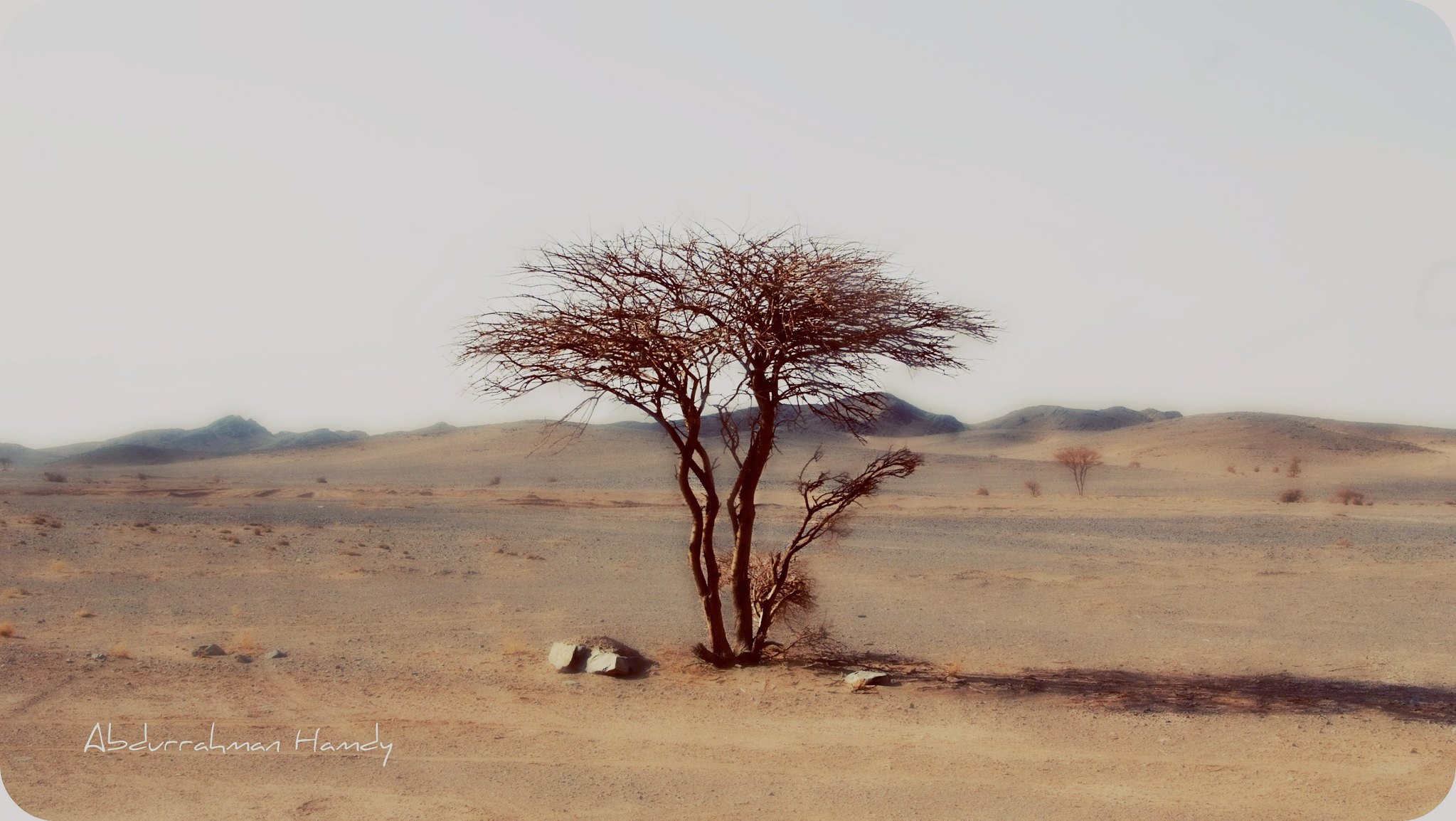The image showcases a striking scene that blurs the line between a photograph and a painting due to its unique lighting. Dominating the center is a leafless tree, its gnarled branches stretching out into the air, suggesting it has weathered many seasons. The setting extends across a mostly flat expanse of dirt or sand, with gentle hills rising towards the background, imparting a sense of depth. Sparse vegetation marks the arid landscape, with only the occasional rock dotting the sandy ground. To the right of the main tree, another similar tree stands further back. The sky above is overcast, infusing the scene with muted tones of gray and white. In the lower left-hand corner, the artwork bears a faint signature—possibly "Abduraman Hardy" or "Handy"—adding a touch of mystery to the creator's identity. The overall ambiance suggests a high desert environment, captured in a moment of stark solitude during midday.